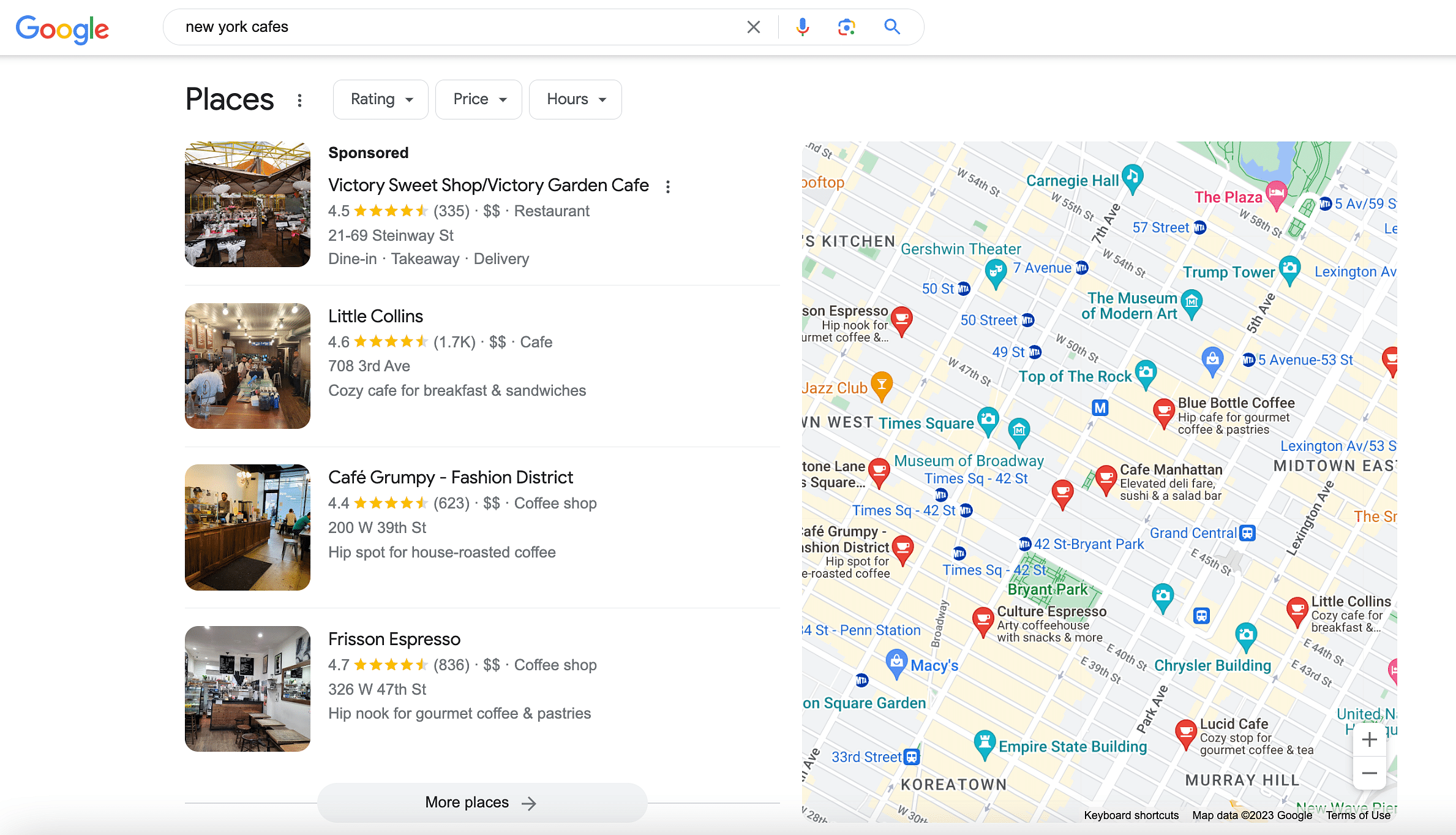The image is a screenshot from Google featuring a search query for "New York cafes." In the upper left corner, the recognizable Google logo is visible, followed by a search bar where the query has been typed. Below the search bar, various filters including 'Rating,' 'Price,' and 'Hours' are available. 

The search results are prominently displayed with the top entry being a sponsored listing for "Victory Sweet Shop/Victory Garden Cafe," which boasts a rating of 4.5 stars based on 335 reviews. The second result is "Little Collins," holding a 4.6-star rating with 1.7K reviews. Next is "Cafe Grumpy in the Fashion District," rated at 4.4 stars from 623 reviews. The final listed cafe is "Fishon Espresso," which has a high rating of 4.7 stars with 836 reviews. Below these results, a "More Places" button invites further exploration.

On the right side of the screen, a map displays numerous location markers corresponding to the cafes listed, providing a geographical context to the search results.